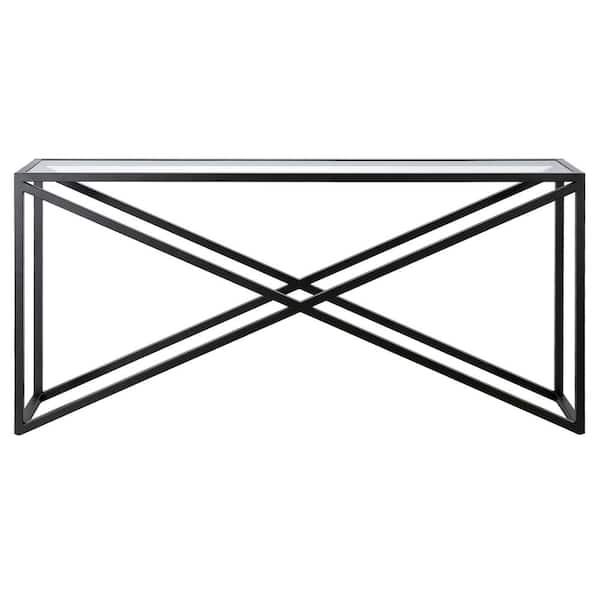This is a photograph of a minimalist coffee table taken from a side view against a completely solid white background with no shadows or other objects. The coffee table features a sleek glass top supported by a black metal frame. The sides of the table have an X-shaped support structure, with dark black diagonal bars intersecting from the bottom left to the top right and from the top left to the bottom right, creating a distinct and sturdy pattern. The short ends of the table are mostly open, except for a single black bar at the bottom for additional support. The table's frame transitions from an off-gray to a metallic black color, enhancing its modern aesthetic. This image captures the table's design from an angle that allows the overlapping X patterns on both sides to be seen clearly.